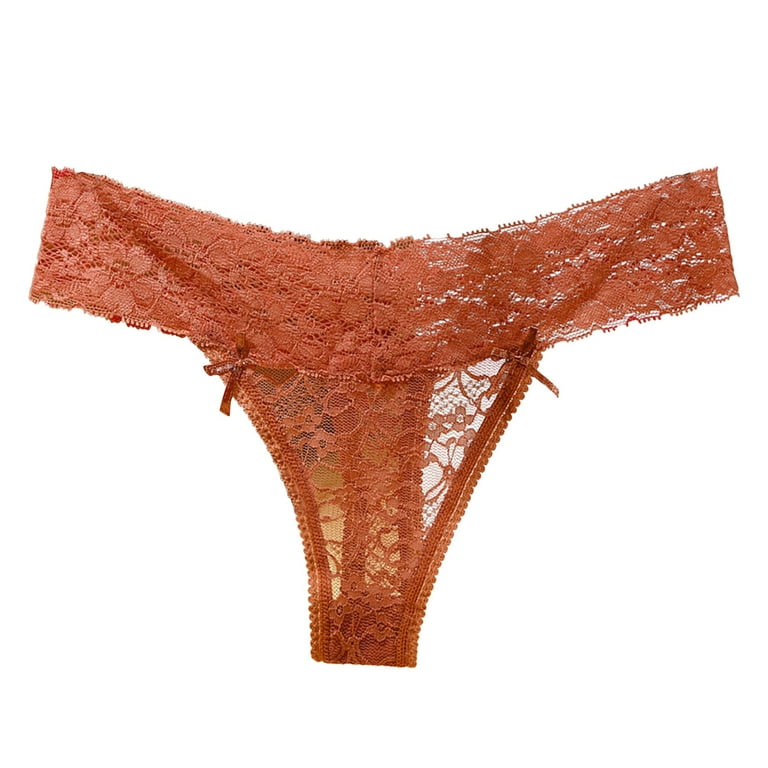The image depicts a pair of medium pink lace thong underwear positioned against a solid white, transparent background. The thong features a prominent elastic lace waistband that curves gracefully from the upper left to the right, dipping slightly in the middle. The main body of the underwear is crafted from nearly see-through, intricate floral lace, allowing a glimpse of the back strip through the front section. On either side of the top of the thong, where the lace meets the waistband, there are small, delicate red bows or ribbons, adding a dainty touch. The material is characterized by its thin, lacy, and decorative nature, suggesting an intimate, sensual design intended to elicit a reaction of sexual arousal. Despite its delicate appearance, the thong is unoccupied, set plainly against the background, highlighting every detailed feature of the garment.